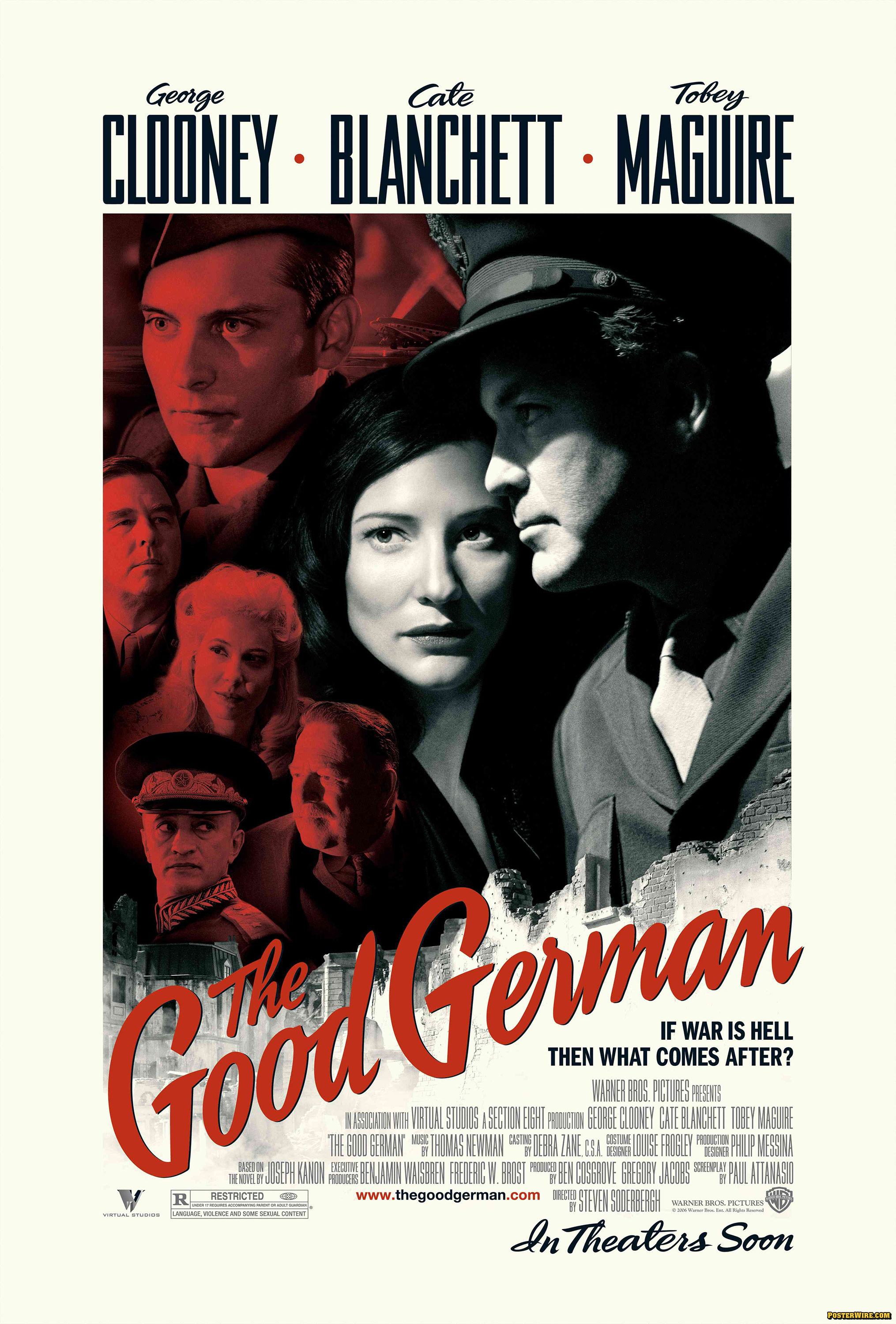This is a photograph of a movie poster for the film "The Good German." The poster primarily features a black-and-white image with selective red tones. Dominating the center is a close-up of a woman with dark hair adjacent to a man's profile, who is attired in a WWII uniform complete with a hat, suit, and tie. The title, "The Good German," is prominently displayed in red text running diagonally from the bottom left corner towards the top right. Underneath the title, in smaller black lettering, is the tagline: "If war is hell, then what comes after?"

At the top of the poster, the names of the stars are listed in black text against a white background: George Clooney, Cate Blanchett, and Tobey Maguire. In the background on the left side of the poster, a series of smaller black-and-white images have a red filter overlay. Among these images, Tobey Maguire is discernible along with other actors, including one wearing a Nazi officer's uniform.

Additional details include a small, illegible text block at the bottom, listing the film's credits and production details. The Warner Brothers logo is also featured, and text on the right side of the poster announces the film's release with, "In theaters soon."